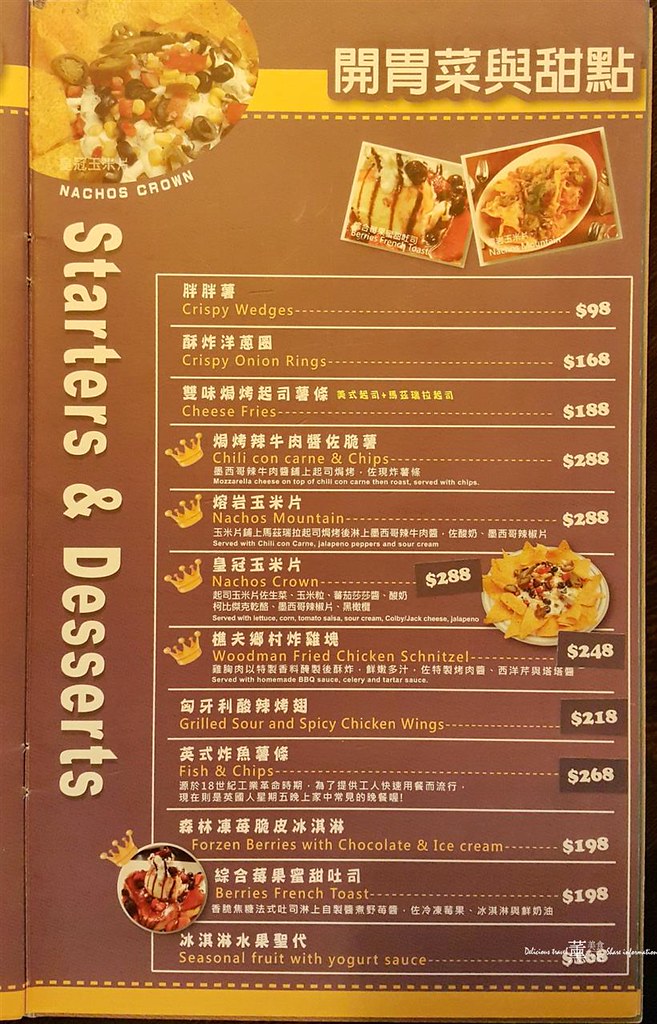The image showcases a restaurant menu presented on a brown-colored paper with a yellow trim and predominantly white text. In the upper left corner, there is a photograph of a dish labeled "Nachos Crown" featuring a large serving of nachos. This picture includes Chinese characters in white and a yellow strip across it. Below this, there are images depicting two other visually appealing dishes. Down the left side of the menu, the sections "Starters" and "Desserts" are listed in white text.

The starters include:
- Crispy Wedges priced at $98
- Crispy Onion Rings for $168
- Cheese Fries at $188
- Chili Con Carne and Chips for $288
- Nachos Mountain priced at $288
- Nachos Crown at $288
- Woodman Fried Chicken Schnitzel priced at $248
- Grilled Sour and Spicy Chicken Wings at $218
- Fish and Chips for $268

The dessert section offers:
- Frozen Berries with Chocolate and Ice Cream priced at $198
- Berries French Toast for $198
- Seasonal Fruit with Yogurt Sauce (price not listed)